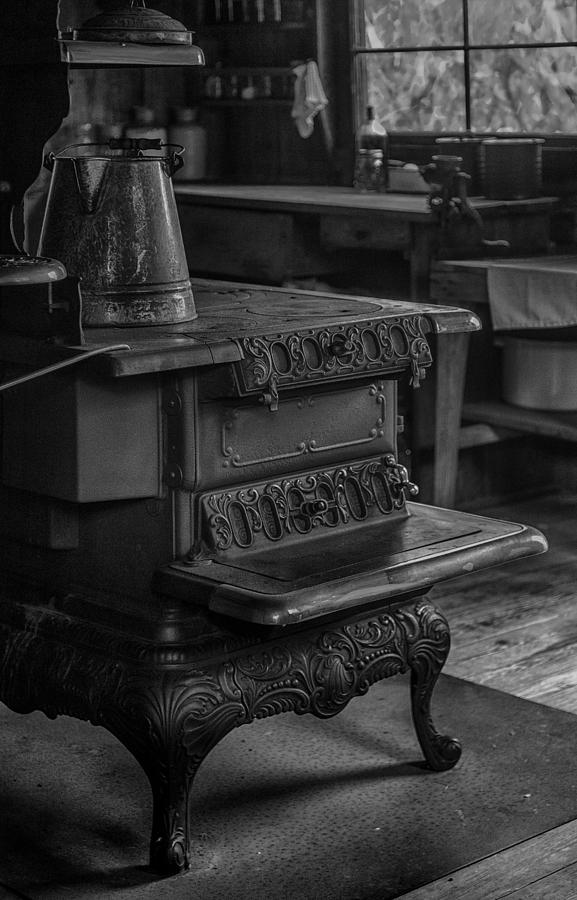This detailed black and white photograph showcases an antique cast iron wood-burning stove, complete with ornate designs and standing on four sturdy legs. The elaborate stove, likely used historically to heat homes, features a side table and space to warm pots on its top surface. Positioned on the stove is a bucket of water. The setting appears to be a kitchen, as indicated by the presence of a countertop with various circular containers and a bottle. A smaller table accompanies a larger table on the right-hand side. The area is grounded by a wooden floor and partially covered with a small black rug in the center. Towards the upper right corner of the image, a window reveals the view outside, adding a touch of natural light to this nostalgic scene.